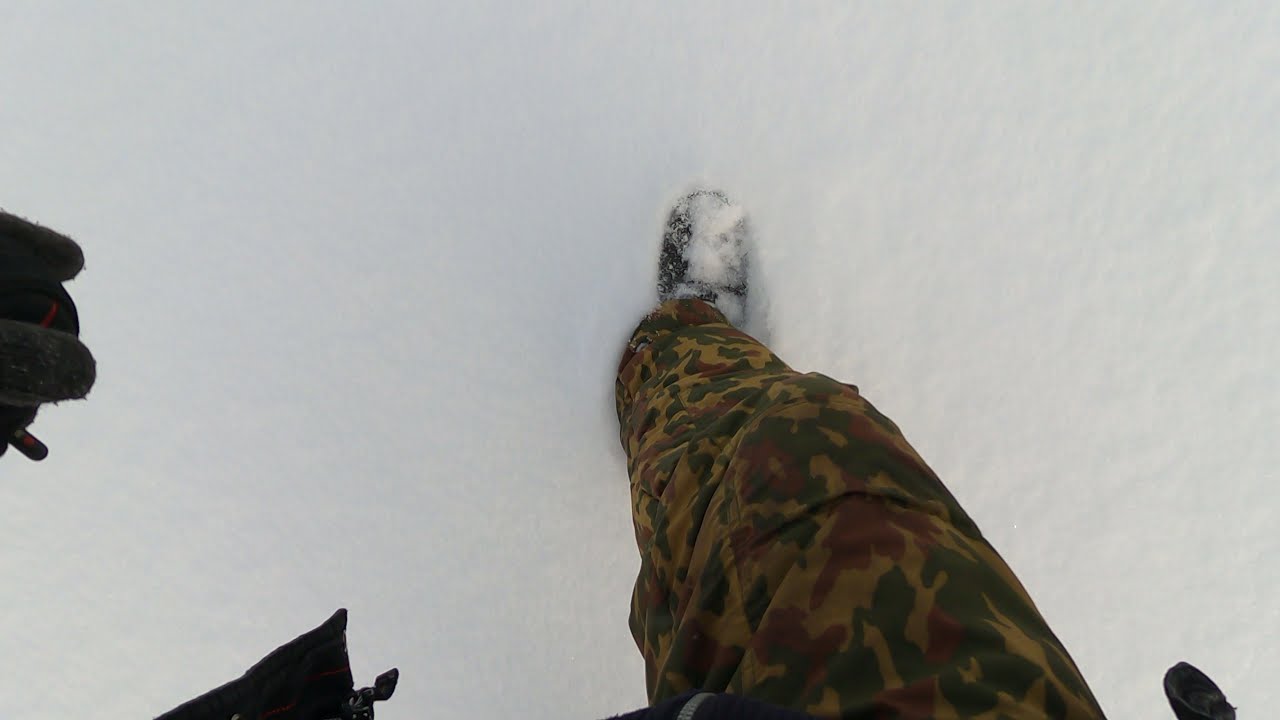This photograph is taken from the perspective of a person looking down at their foot as it sinks into pristine white snow. The ground is covered in snow that appears untouched, with a slight shadow on the left side. The person is wearing black boots, mostly obscured by powdery snow, making it difficult to see details. They are dressed in camouflage pants featuring a mix of tan, dark brown, and olive green colors. A glimpse of their gloved hand and what appears to be the black hem of their coat or jacket is visible in the lower left corner of the image. The snow on the right side of the foot appears brighter, hinting at the direction of the light source.